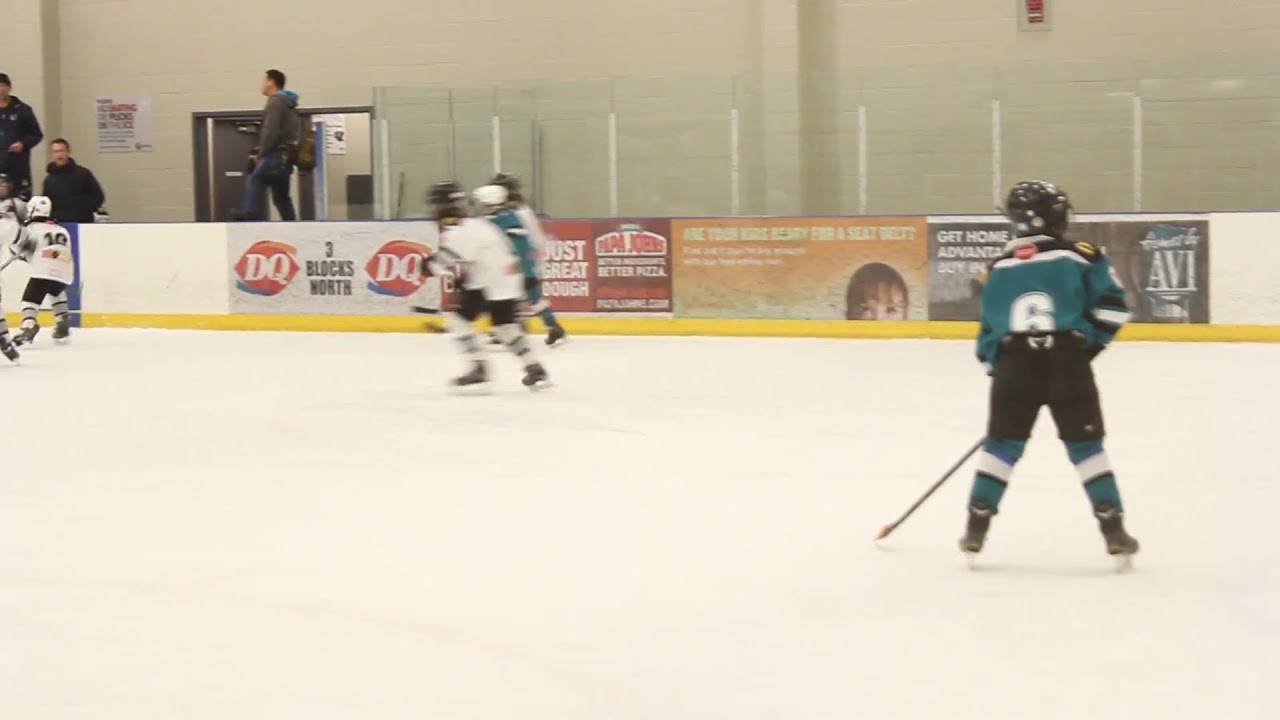This detailed image captures an indoor ice rink during what appears to be a peewee hockey game featuring two teams of young players, likely aged 10 to 12. The rink's ice surface, surrounded by barriers, hosts several hockey players wearing full protective gear and helmets. The players, identifiable only by their uniforms, are mostly seen from the side or back, obscuring their faces. One team sports turquoise and black jerseys, while the other team is in white and black. Specific players can be noted, such as number 6 from the turquoise team and number 10 from the white team.

The rink's walls are adorned with various advertisements, including notable ones for Dairy Queen and Papa John's. The Dairy Queen (DQ) ad features a distinctive oval logo with italicized white letters. The Papa John's ad showcases their red font logo along with their slogan "Better Ingredients, Better Pizza." Additional ads are present, including one mentioning a seatbelt, but they are less clear.

Given the detailed descriptions of the uniforms, the presence of full gear, and the barrier advertisements, the image likely depicts a mid-game scenario during a youth hockey tournament, set around midday. The vibrant colors in the scene include white, blue, black, red, yellow, orange, turquoise, and gray, with parents possibly watching from the sides, engrossed in the spirited match.